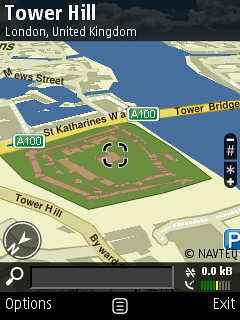This image is a screenshot of a map focusing on Tower Hill, London, United Kingdom. The top of the image features a black banner with white text indicating the location. The map itself displays an area of land on the left and a dark blue body of water on the right, separated by a yellow line representing the Tower Bridge, labeled with "St. Catharines W" and "A100." Directly below this bridge is a rectangular grassy area with brown patches, possibly a park, highlighted by a zoom-in graphic. The map also includes a small, gray compass pointing north in the bottom right corner, as well as options to zoom in and out on the right side. The bottom of the image features another black banner with a search bar, magnifying glass icon, and buttons labeled options, menu, and exit.